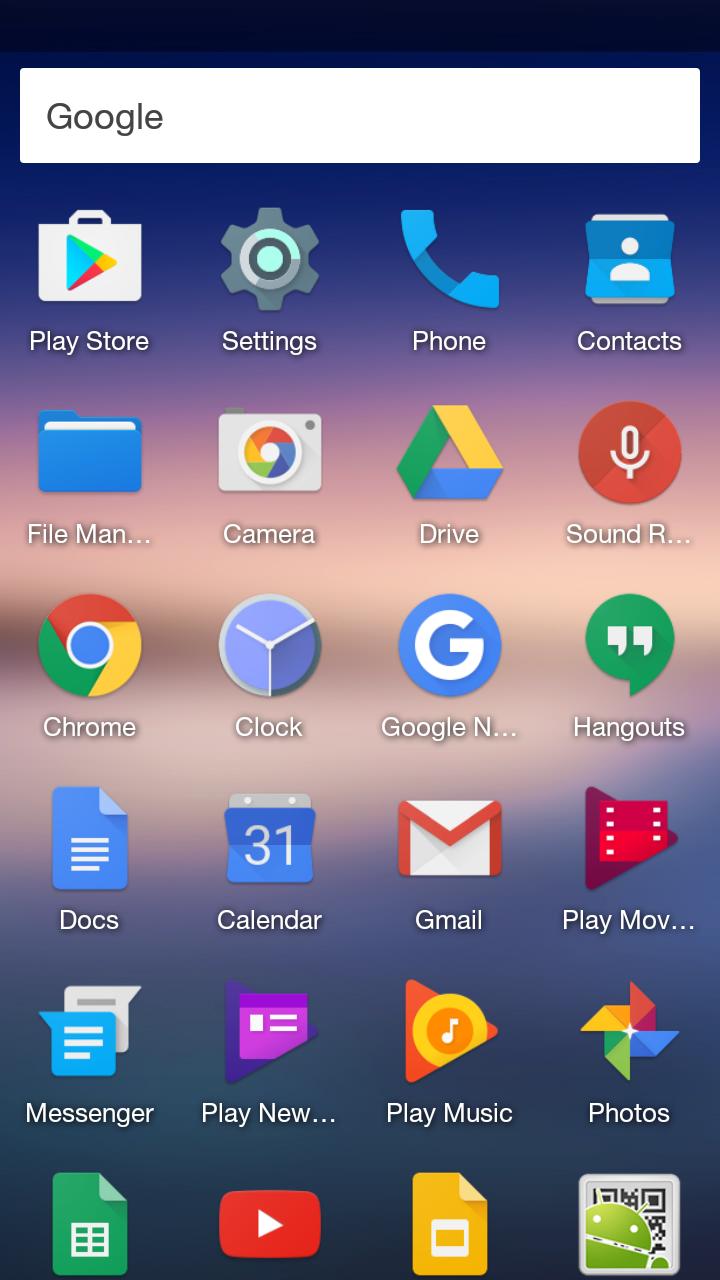**Detailed Caption:**

The screenshot depicts the home screen of an Android phone, presenting a range of application icons neatly arranged. At the top, there's a search bar, followed by an array of app icons. Featured prominently are:

1. **Play Store** (represented by a shopping bag)
2. **Settings** (gear icon)
3. **Phone** (phone icon)
4. **Contacts** (address book icon)
5. **File Manager** (file folder icon)
6. **Camera** (camera icon)
7. **Drive** (triangle icon)
8. **Sound Recording** (microphone symbol)
9. **Chrome** (Google Chrome logo)
10. **Clock** (clock icon)
11. **A partially visible Google app** starting with N (cut off with the Google 'G' logo)
12. **Hangouts** (quotation marks in a speech bubble)
13. **Docs** (document icon)
14. **Calendar** (calendar icon)
15. **Gmail** (envelope icon)
16. **Play Movies** (play button and a piece of film)
17. **Messenger** (two message bubbles)
18. **Play New...** (cut off, possibly Play News, with a play button and another symbol)
19. **Play Music** (play button with a musical note)
20. **Photos** (colorful pinwheel icon)

Along the bottom, there are additional symbols, which include but are not clearly named due to visibility restrictions. These appear to include:

1. **Documents icon**
2. **YouTube** 
3. **An unidentified yellow icon**
4. **QR code reader**

These elements create a typical and functional layout for easy access to commonly used applications on the device.